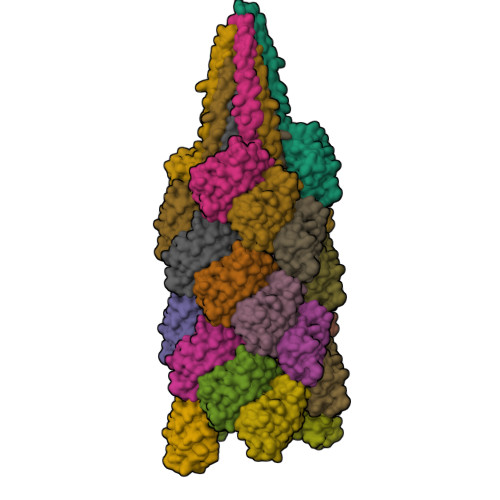The image depicts a lumpy, cone-shaped structure composed of various colored segments that create a patchwork appearance. The structure appears roughly textured and features segments of brown, pink, green, gray, and purple. The brown color dominates the left side, transitioning to pink in the center, and green on the right side, with gray and purple patches emerging toward the lower part of the structure. The overall form vaguely resembles a person standing upright, with discernible head, body, and legs formed by these multicolored, bumpy segments.